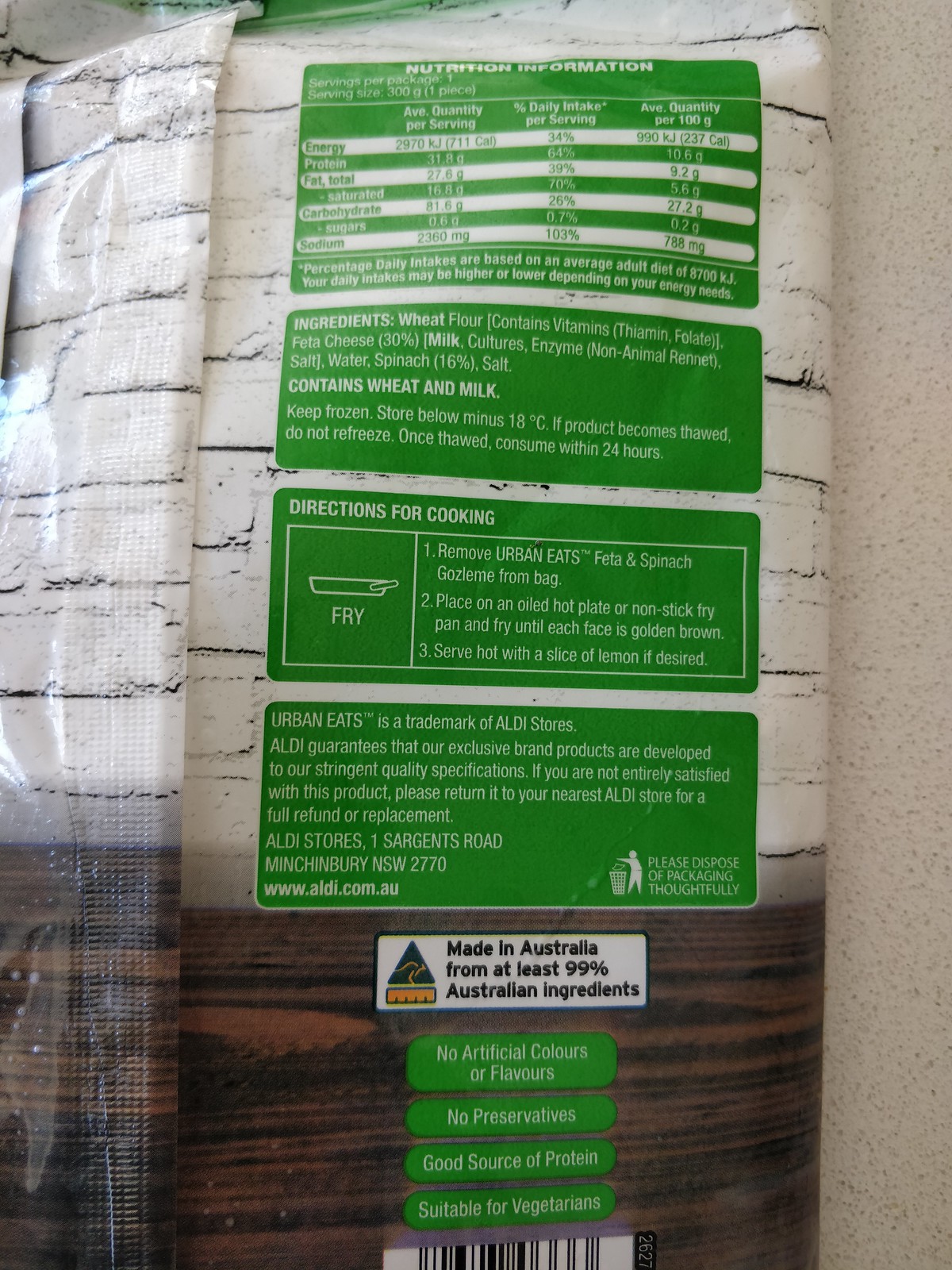This image depicts the back of a food package, specifically positioned on a white, speckled linoleum surface. The packaging is visually striking with its two-toned design: the top portion features a pattern mimicking white outdoor paneling, while the bottom showcases a wood grain texture. At the top of the bag, there's an eye-catching green nutrition label with white font, prominently displaying "Nutrition Information." We're given a close-up view of the detailed chart that follows, although it's somewhat difficult to discern. Below the nutrition information, a list of ingredients begins with "wheat flour" and "milk," continuing with other components. Further down, there's another green label titled "Directions for Cooking," which instructs the user to remove the "Urban Eats Feta and Spinach Gazette" from the bag and suggests frying as the method of preparation.